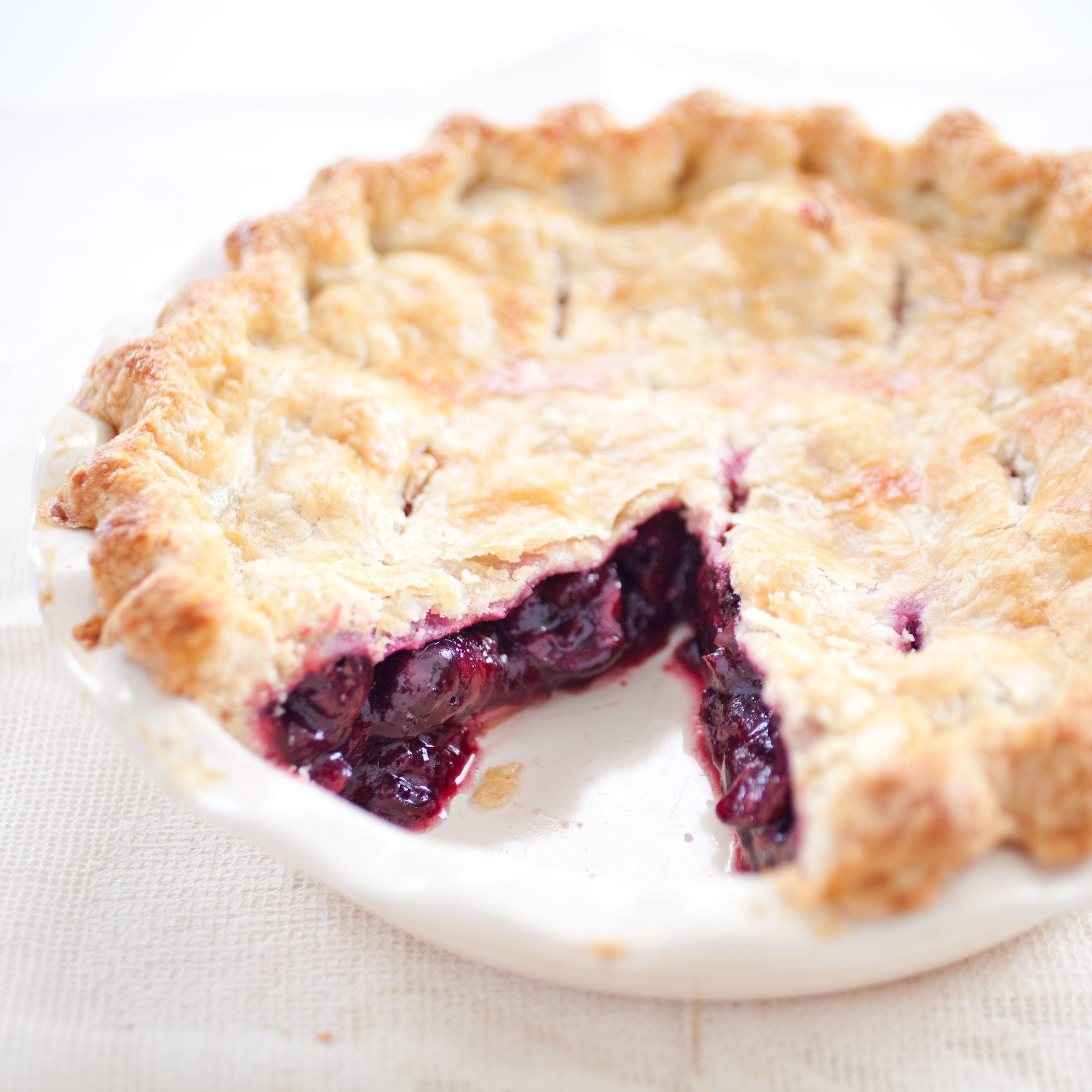The square photograph features a close-up of a large, homemade pie with a golden crust, placed in a round, white porcelain pie dish. The pie has a triangular slice missing, allowing a clear view of its rich, syrupy blueberry filling, which appears deep purple in color with visible pieces of blueberries. The crust is scalloped along the edges and marked with various slits for steam release. The pie dish sits on a flat surface covered with a white kitchen towel featuring a faint crisscross pattern. Scattered pie crumbs add to the authentic homemade appeal, with the detailed focus accentuating the pie's delectable texture and filling, making the rest of the image gently fade out of focus.